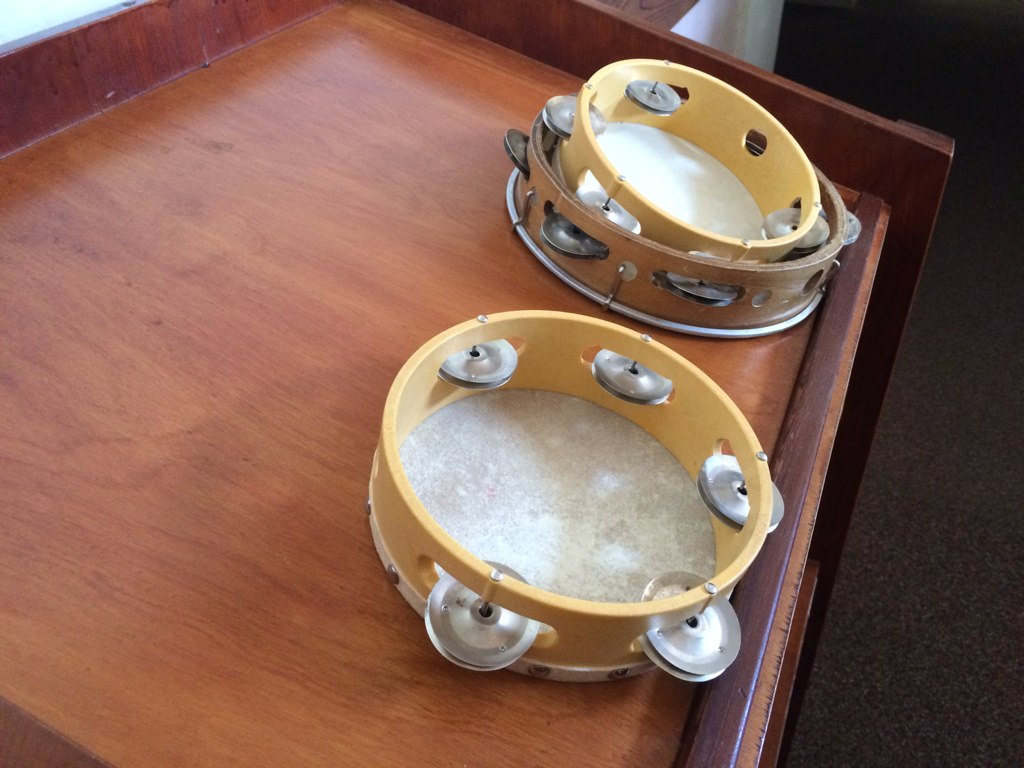The image portrays a total of three tambourines carefully arranged within a wooden drawer or tray, which has a lip to prevent them from falling out. The drawer is made of medium brown wood, possibly cherry, and is positioned against some cabinetry with visible brown carpet in the background. 

On the left side of the drawer lies a large tambourine, turned upside down, showcasing five pairs of metal cymbals. To its right rests another large tambourine, slightly darker in wood tone. Nested inside this darker tambourine is a smaller one, also upside down but of a lighter color similar to the tambourine on the left. The space above the tambourines is open, revealing the interior of the drawer. The scene is detailed with wooden cabinet structures nearby, adding an extra layer of context to the setting.